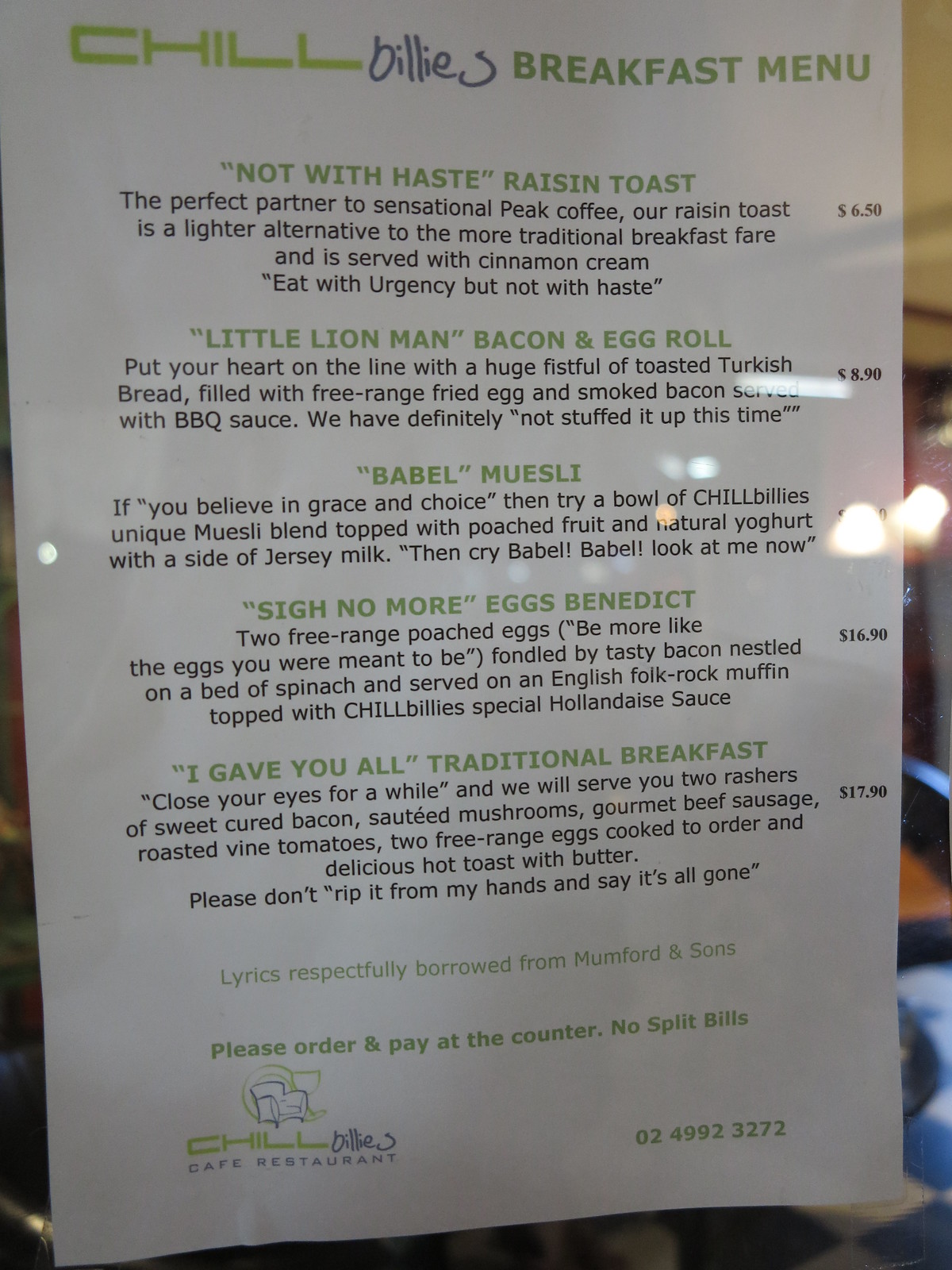A photograph of Billy's Restaurant menu titled "Chill Billy's Breakfast Menu" is shown. The phrase "Chill Breakfast Menu" is elegantly displayed in green font, while "Billy's" is in a distinct black font, making it stand out. The white menu paper features a list of unique breakfast options, all themed with names inspired by Mumford and Sons lyrics, with descriptions and prices detailed in black text beside each item.

The first item, "Not With Haste Raisin Toast" cost $6.50 and is served with cinnamon cream, suggested as a perfect partner to Sensational Peak Coffee. The description whimsically advises, "Eat with urgency, not with haste."

The next item is "Little Lion Man Bacon and Egg Roll" priced at $8.90. It includes free-range fried egg and smoked bacon in toasted Turkish bread, topped with barbecue sauce. The menu jokingly reassures, "We have definitely not stuffed it up this time."

Other intriguing selections include "Babble Moose Sly" and "Sigh More Eggs Benedict." The last option is "I Gave You All Traditional Breakfast," each item adhering to the lyrical theme.

At the bottom of the menu, a footnote reads: "Lyrics respectfully borrowed from Mumford and Sons. Please order and pay at the counter. No split bills." Additionally, there’s a restaurant logo and a phone number, 024 9923 272, adding to the authenticity. The background of the photograph is blurry, emphasizing the menu's detailed design.